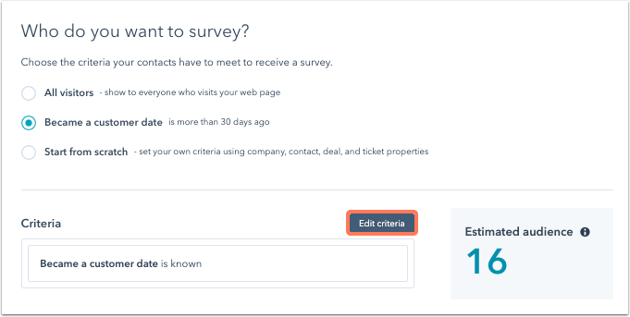The image displays a section of a survey setup interface on a predominantly white background. The layout is horizontal in orientation rather than vertical. At the top, in a gray font, a question reads: "Who do you want to survey?" followed by instructions in lighter gray, "Choose the criteria your contacts have to meet to receive a survey."

Below this, two options are presented. The first option, "All visitors," is in bold black font and is accompanied by a white circle checkbox. This option indicates that the survey will be shown to everyone who visits the webpage. 

The second option, "Became a customer date is more than 30 days ago," is distinguished with a bold font and a blue dot next to it. 

Further down, there's an option titled "Start from scratch," also in bold font, which allows users to create custom criteria using company contacts, deals, and ticket priorities.

Underneath, a subsection labeled "Criteria" includes a specific criterion, "Became a customer date is known," alongside an "Edit criteria" button in blue font with an orange border. The section also provides an estimated audience count, marked by the text "Estimated audience" and an information icon. The number "16" is displayed beneath this text in blue.